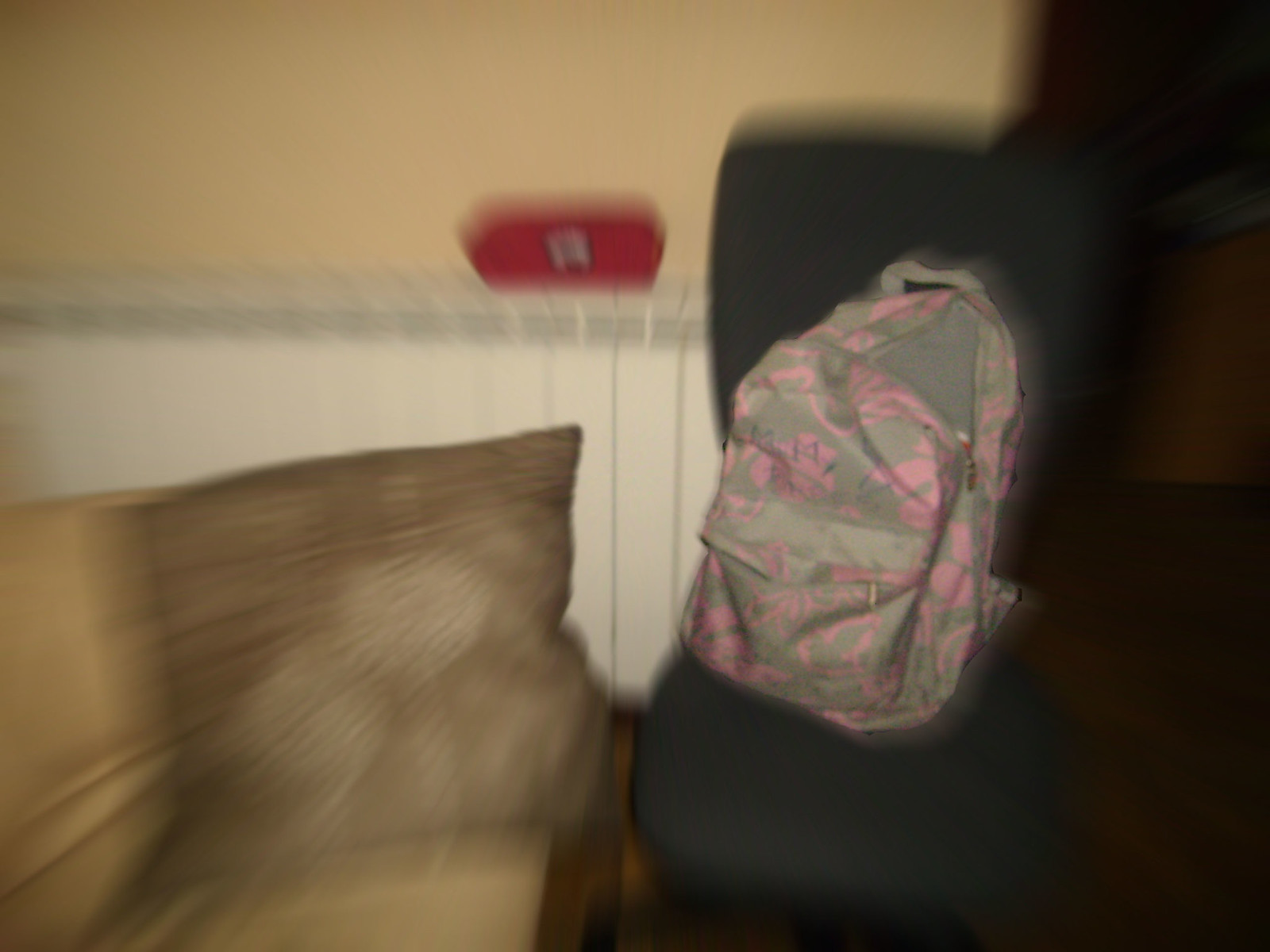This image is a very blurry color snapshot likely taken with a low-quality instant camera, depicting a room interior. A prominent feature is a gray and pink backpack situated near the center-right of the image, leaning against a dark object, possibly a couch or chair. The backpack appears to have multiple compartments with zippers and some indistinct writing or designs in blue pen. To the left, there is a dark yellow or light brown couch with a brown throw pillow. The background features a light yellow wall with white wooden baseboard trim and a noticeable red object between the wall and the trim. Due to the significant motion blur, many details are hard to discern.